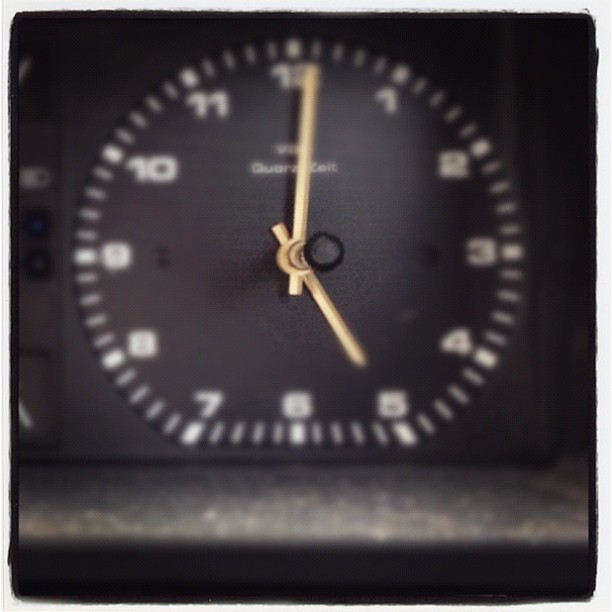This close-up color photograph captures an analogue clock face, likely from a vintage car dashboard. The clock’s hands, an off-white beige or metallic gold color, stand prominently in focus while the numbers around the dial are blurry and indistinct. The minute hand reads 1 minute past the 12 o'clock position, and the hour hand points to the 5, indicating the time as 5:01. A small black adjustment knob protrudes from the center, attached to a rod running through the clock hands, reminiscent of older vehicle clocks where time is manually set from the front. The clock is encased in a black panel, potentially made of plastic, and likely covered by translucent plastic or glass. Beneath the 12, a word is faintly visible, though not clearly readable. The contrast between the focused hands and blurred numbers adds depth to the image, highlighting the intricate details of the clock face against its predominantly black encasement.